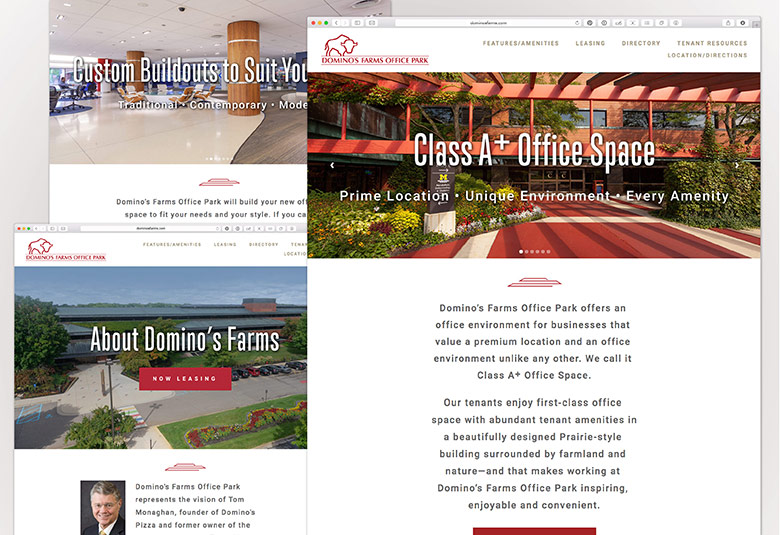The image is a busy screenshot featuring several pages overlaid on top of each other, set against a light gray background. The largest and most prominent of these pages is positioned nearer to the right side of the screenshot and has a vertical orientation. This page is dedicated to Domino's Farms Office Park and prominently displays a series of headings on the right, including "Features and Amenities," "Leasing," "Directory," "Tenant Resources," and "Location Directions." Below these headings is a large horizontal rectangular box showcasing the exterior of an office space, with lush greenery and a rust-colored building. The image within the box is overlaid with white text that reads: "Class A+ Office Space. Prime Location, Unique Environment, Every Amenity."

On the lower left of the screenshot, there is evidence that the link titled "About Domino's Farms" has been clicked, revealing a section beneath it with a box that states "Now Leasing." The topmost page is partially obscured by the other two, making much of its content difficult to discern, but it appears to display the interior of an office building. This section features text highlighting customizable office buildouts, with options described as "Traditional, Contemporary, Modern."